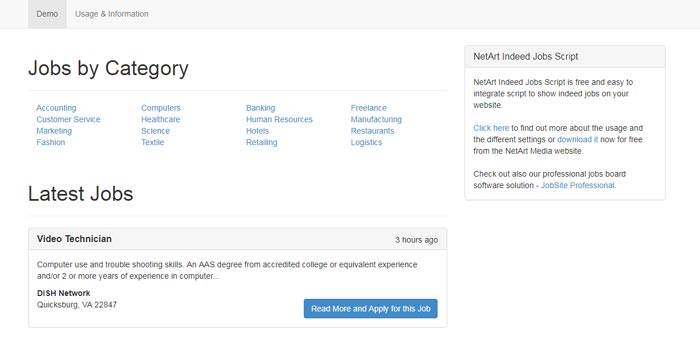In the top left corner of the webpage, there is a heading that reads "Demo," highlighted in light gray and written in unbolded black text. To its right, set against a light gray background, is the label "Usage & Information," with the ampersand sign used to connect the words.

The main section of the webpage features a clean, white background. On the left side, there is a black header titled "Jobs by Category." Below the header, a thin, light gray line acts as a divider. Underneath, various job categories are listed in blue text, signifying that they are clickable links. The categories include:

- Accounting
- Customer Service
- Marketing
- Fashion
- Computers
- Healthcare
- Science
- Textile
- Banking
- Human Resources
- Hotels
- Retailing
- Freelance
- Manufacturing
- Restaurants
- Logistics

Adjacent to this section on the right side, there is a square pop-up window. It features a light gray heading with the black text "NetArt Indeed Jobs Script." The interior of the pop-up has a white background with additional black text that reads: "NetArt Indeed Jobs Script is a free and easy-to-integrate script to show Indeed jobs on your website." Within the text, "Click here" is shown in blue, indicating that it’s a clickable link providing more information about usage and settings, or for downloading the script. The phrase "Now, for free from the NetArt Media website" appears next, followed by "Check out also our Professional Jobs Board Software Solution-Jobsite Professional," also highlighted in blue and clickable.

Under the "Jobs by Category" header, there's another black-text heading saying "Latest Jobs." Below this, a pop-up job listing for a "Video Technician" is displayed. To the right of the job listing is a blue rectangular button with white text that reads "Read More and Apply for this Job."